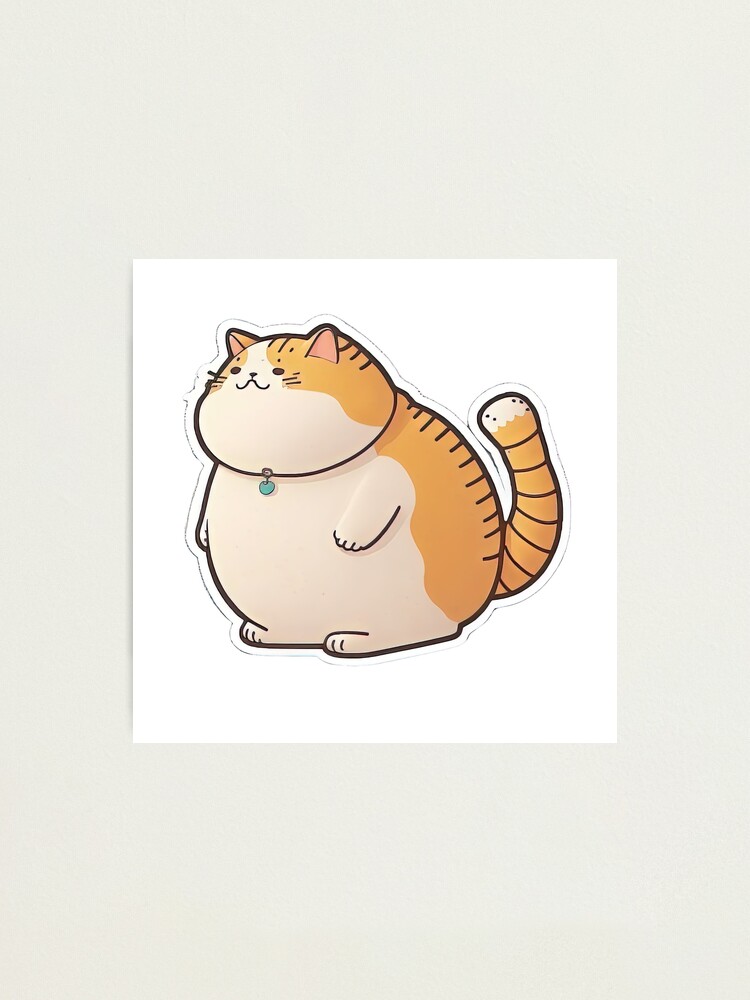The image shows a digital illustration of an extremely overweight, cartoon-like cat that appears to be a sticker positioned on a white square of paper, bordered by a gray piece of paper. The fat cat's round, large face features pink ears, visible eyes, whiskers, a nose, and a mouth, while a string collar dangles a light blue, heart-shaped pendant under its chin. The cat's body is divided into sections of color: its front face and underbody are white, transitioning to a ginger back with black stripes, and an orange tail with black stripes that ends in a white tip with black dots. The cat's limbs are barely visible due to its size, and its facial expression conveys happiness.